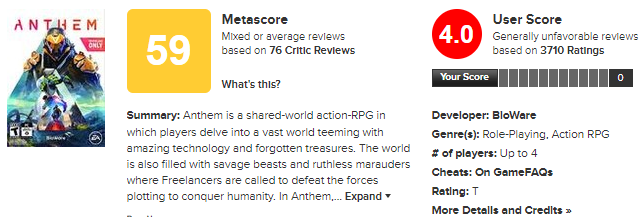Here is a cleaned-up and detailed caption for the image based on the provided voice description:

---

A detailed screenshot from a video game review site features the game Anthem. On the left side, there is the official game box art, prominently displaying the title "Anthem" in bold black letters. The cover showcases a powerful character clad in striking red, yellow, gold, and white armor, epitomizing the game's vibrant aesthetics.

Next to the box art is a yellow square with the number '59' in white, indicating the Metascore, a measure reflecting 'Mixed or average reviews based on 77 critic scores.' Below the Metascore is a summary of Anthem, which describes it as a shared-world RPG where players explore a vast, technologically advanced world filled with forgotten treasures, savage beasts, and ruthless opponents. Players, known as freelancers, take on the challenge of defeating forces that threaten humanity.

Further details include a red circle displaying a '4.0' user score in white, signifying 'Generally unfavorable reviews based on 3,710 ratings.' The screenshot indicates the user has not yet rated the game, with their score showing as '0.' Additional game information lists Bioware as the developer, the genre as Role Playing (RPG), the game supports up to 4 players, and there are cheats available on GameFAQs. The game has a 'T' rating, and a prompt for more details and credits is indicated by two arrows pointing to the right.